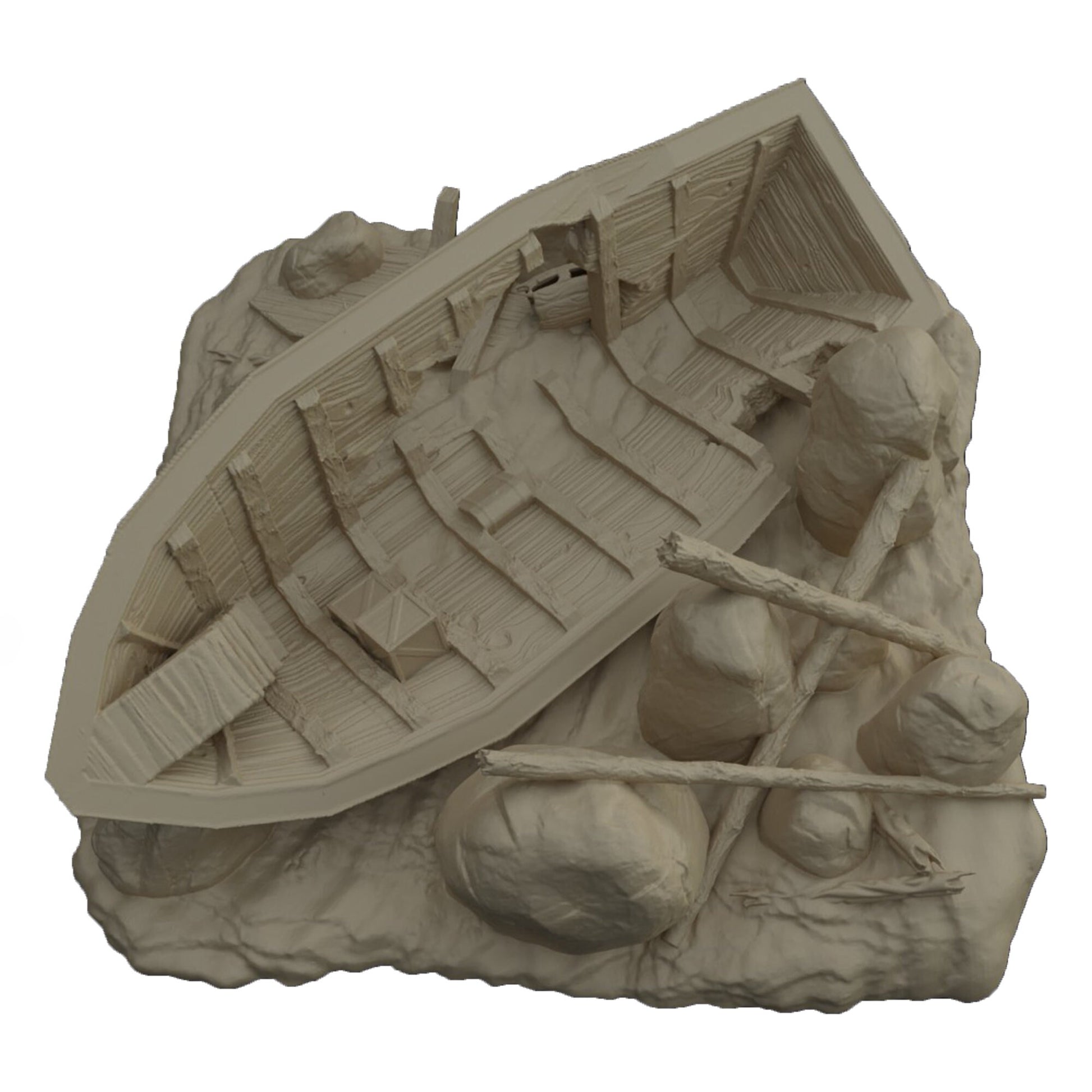This image captures a detailed 3D-printed sculpture of a wrecked rowboat, viewed from a top-down perspective and set against a largely white, digitally edited background. The square-shaped frame contains an intricately designed miniature scene, meant to emulate a shipwreck on the ocean floor. The central focus is the shattered boat, with a triangular bow positioned in the lower left and a flat stern in the upper right. The top decks have decayed, exposing the ship's interior littered with crates and chests. Surrounding the wreck are clusters of textured, round rocks and three broken masts resembling tree branches, enhancing the scene's sense of destruction and abandonment. The sculpture, primarily brown in color, is a testament to the creator's skill, expertly crafted to mimic a haunting yet captivating underwater shipwreck tableau.